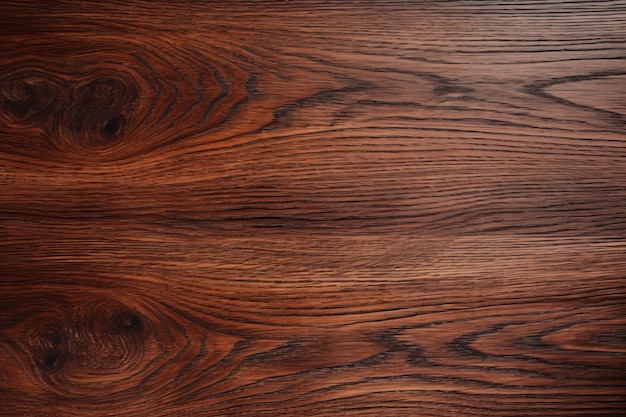The image depicts a close-up view of two polished and stained wooden planks, which might be part of a flooring or a table. The wood features a rich combination of brown, light brown, dark brown, and dark cherry reddish hues. The planks exhibit several distinctive black markings that appear predominantly at the top and bottom, forming wave-like patterns. On the left side of the image, there are notable swirling knots, which darken towards their center, creating a focal point. A black line runs horizontally between the two sets of swirls. The surface of the wood is well-trimmed and polished, highlighting its natural grain and texture. The detailed staining and the seamless blend of colors suggest a refined craftsmanship, enhancing the aesthetic appeal of the wood.